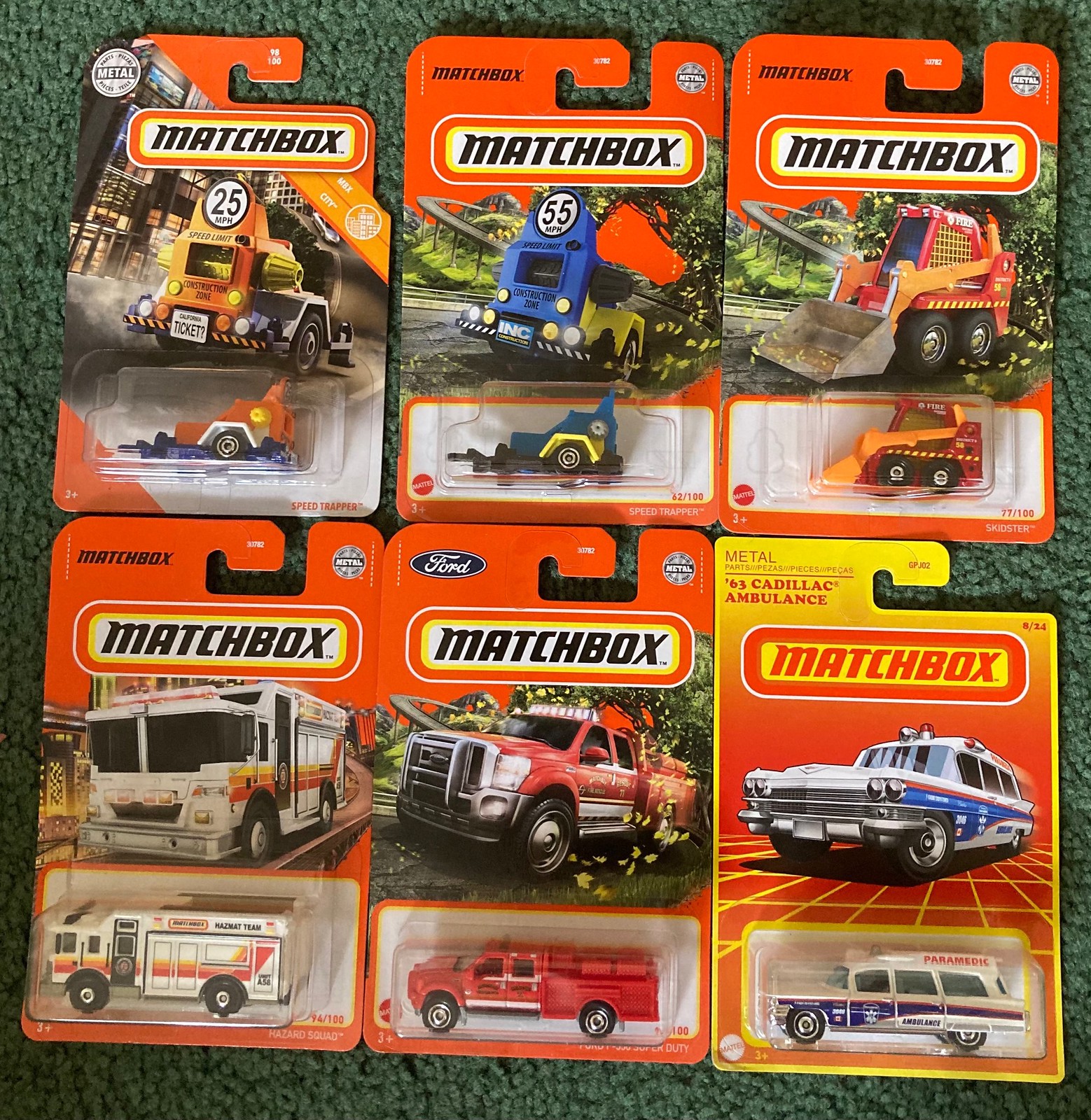This photograph showcases a neatly arranged collection of six Matchbox model scale cars, all in their original, mint condition packaging. The packages are laid out on a green carpet in two rows of three, with three cars along the top row and three along the bottom row. Each package features the classic Matchbox logo at the top, with a white rectangle and black text, though the logo on the bottom right packaging is different, suggesting it is from a unique set or edition.

The cars are clearly visible through the vacuum-formed plastic covers that hold them to their respective cardboard backings. Detailed illustrations of the cars adorn the middle of each package, and the cars are color-coded in a variety of hues. The bottom row consists of emergency vehicles: an ambulance on the left, a fire truck in the middle, and a 63 Cadillac Ambulance labeled "paramedic" on the right. Meanwhile, the top row appears to be construction vehicles, including a red truck labeled "25 MP" and "construction zone," a blue and yellow car marked with "55 MP," and a red bobcat with yellow accents.

This image, with the pristine state of the packaging and organized layout, suggests it may have been taken to showcase the collection for potential sale or to display the collector's pride in preserving these iconic toy cars.